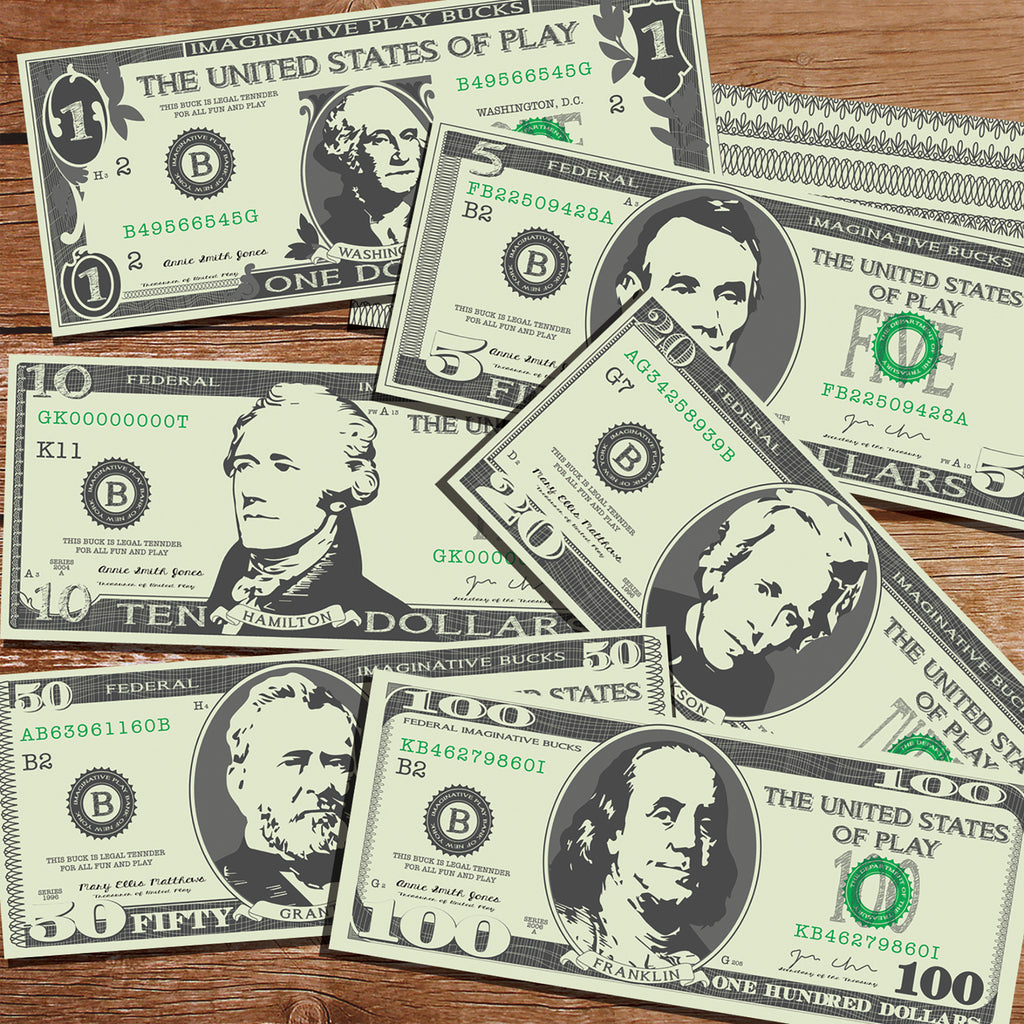The image features a collection of play money, meticulously arranged on a wooden table. The denominations on display are $1, $5, $10, $20, $50, and $100 bills, with the $100 bill positioned at the top. Each bill prominently showcases the phrase "Imaginative Play Bucks, The United States of Play," and bears a striking resemblance to real U.S. currency. The designs include images of historical figures commonly found on actual money: George Washington on the $1 bill, Abraham Lincoln on the $5 bill, Alexander Hamilton on the $10 bill, Andrew Jackson on the $20 bill, Ulysses S. Grant on the $50 bill, and Benjamin Franklin on the $100 bill. The thicker paper and the educational purpose of these bills—likely intended for teaching children about money and counting—affirm their authenticity as play money. Despite their cartoon-like appearance, the attention to detail in both the design and the replication of currency elements offers a convincing simulation of genuine American money.